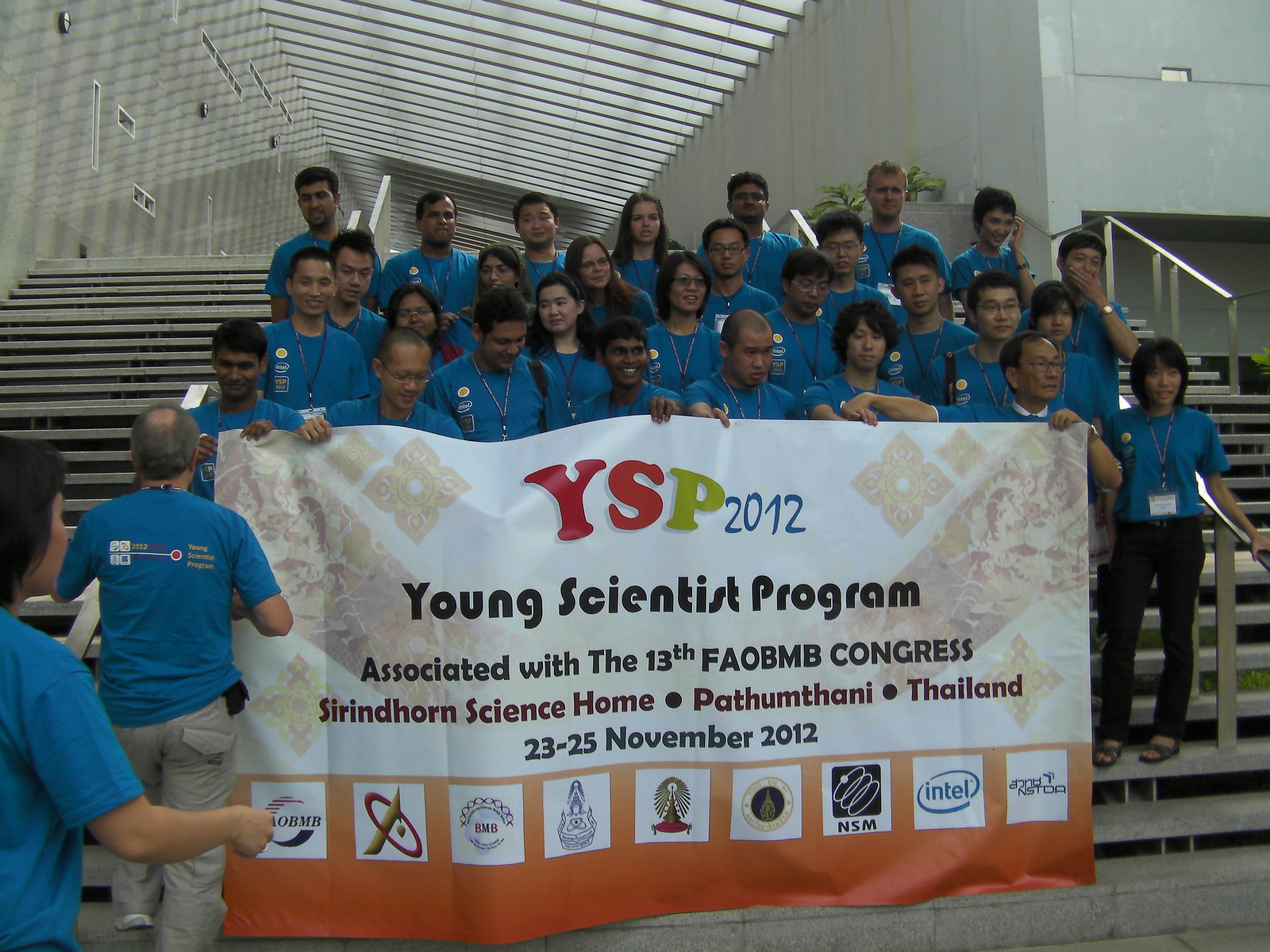This image is a group photo taken on the steps of a modern building featuring an open roof with sunlight filtering through slats. The group, predominantly of Thai descent, includes both men and women, possibly of Indian descent as well, all wearing matching blue T-shirts adorned with the company logo on the chest and text on the back. Some individuals also have lanyards. They are arranged in five rows and are holding a large banner that reads "YSP 2012" in red, green, and blue letters. Below that, in black text, it says, "Young Scientist Program associated with the 13th FAO BMB Congress, Sirindhorn Science Home, Pathum Thani, Thailand, 23-25 November 2012." Various sponsor logos, including those of Intel and NSM, are displayed along the bottom of the banner. One woman on the far right stands out, wearing black slacks.